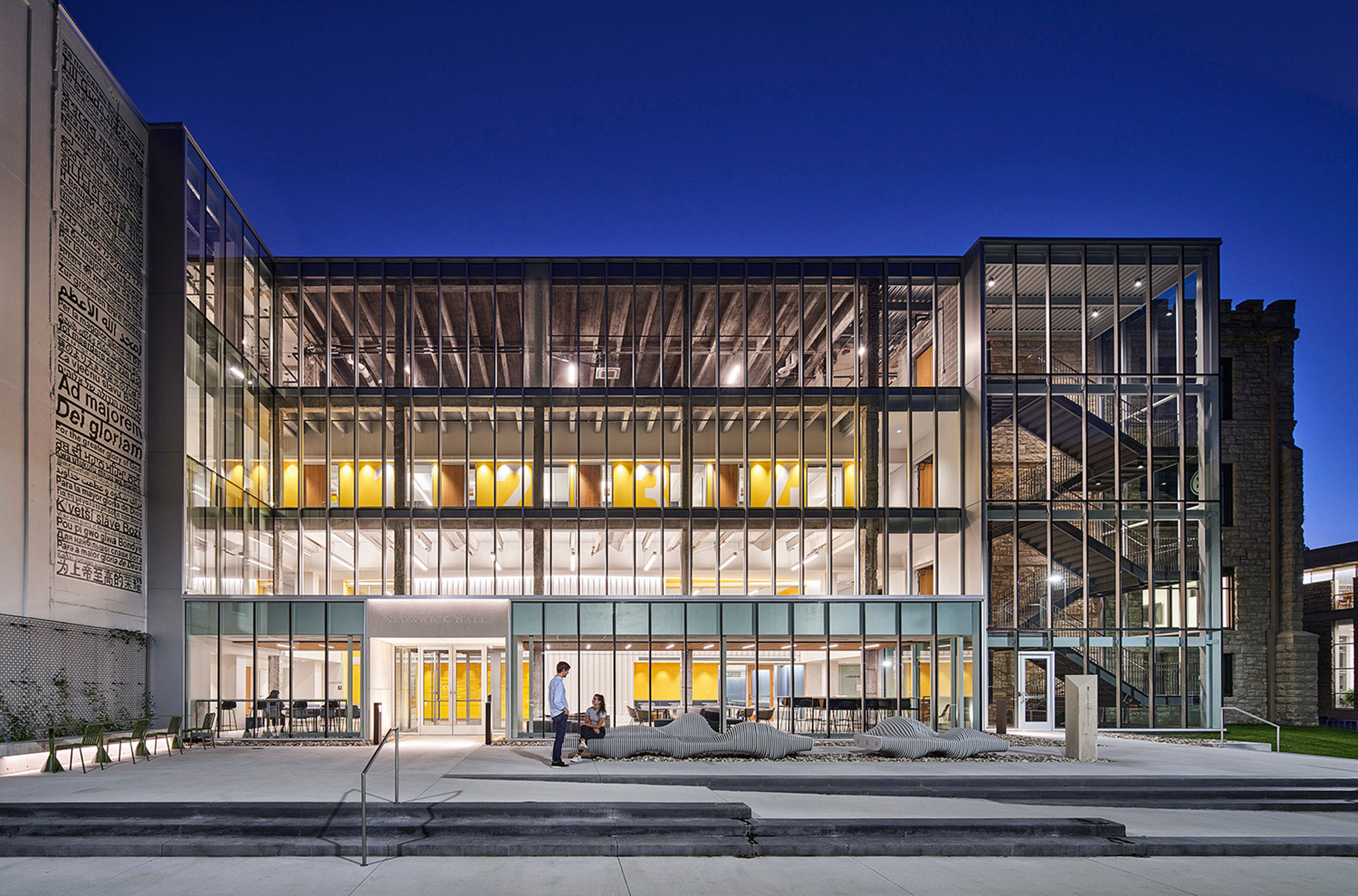This color photograph captures a very large, four-story office building with an elaborate and modern design. The building's facade is primarily made up of expansive glass walls, allowing clear visibility into its interior. The outside view showcases numerous windows and doors, with the interior dramatically lit up, casting a warm yellow glow that contrasts with the dark blue, nighttime sky.

At the entrance of the building, there are several steps leading up, accompanied by a handrail. In front, there's a concrete area furnished with modern sculptures, tables, and chairs. A young woman, dressed in a white blouse and black pants, is seated on one of the chairs, conversing with a young man standing beside her, who is wearing a light blue shirt and dark jeans.

On the right side of the building, a striking section features a glass wall through which you can see a series of staircases backed by a stone wall. Adjacent to the building, there's a large billboard or poster adorned with numerous words in different languages, including the phrase "ad majorum del glorium," though much of the text is not legible from this angle.

Inside the ground floor, there are numerous tables and chairs visible, suggesting it may serve as a communal or dining area. The upper floors are less distinct, primarily showing the ceilings and hinting at a more closed-off or private space. This scene encapsulates a blend of architectural sophistication and a vibrant, urban atmosphere.